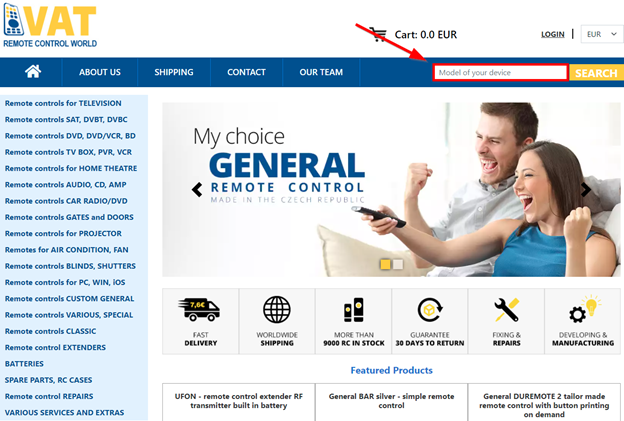The screenshot features the desktop-sized view of a website named "V-A-T Remote Control World" (possibly pronounced VAT). The left side of the page displays a comprehensive menu listing various categories of remote controls, including options for television, DVD, home theater, gates and doors, projectors, air conditioning, blind shutters, and specialized and classic models, offering a wide range of remote controls for different needs. 

Dominating the center of the page, the hero section showcases "My Choice - General Remote Control," which is manufactured in the Czech Republic. This section includes an image of two people enthusiastically using a remote control, their expressions filled with joy and satisfaction.

Below this, there is a list of featured products: the "UFON Remote Control Extender," "General Bar Silver - simple remote control," and the "General Dura Remote," which is described as a durable, tailor-made remote control with customizable button printing options, reflecting the website's diverse and innovative product offerings.